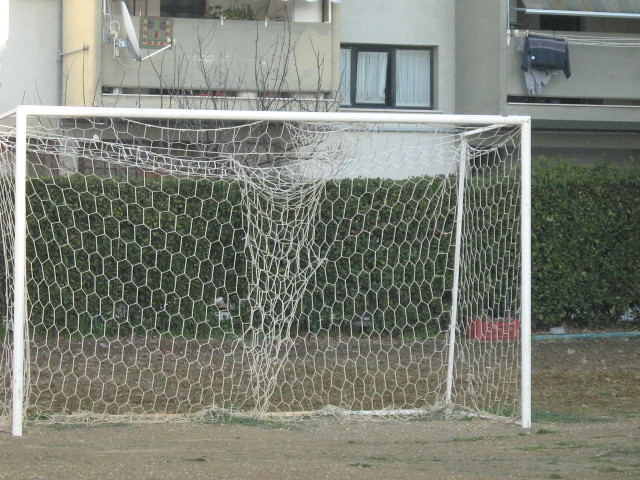A white goal net, somewhat worn and torn from frequent use, stands on a field characterized by patchy grass and dirt. This field is bordered by a well-trimmed green privacy hedge approximately 5 feet tall. Behind the hedge is a residential area featuring a white apartment building. The building has enclosed cement balconies, two of which are visible with one situated in the left and another in the right upper corner. Clothing is seen hanging from the balcony on the right. Additionally, three rectangular windows are positioned between the balconies. The middle of the goal net is notably damaged. The backdrop of the scene includes satellite TV dishes and more balconies, suggesting a heavily frequented and lived-in residential space.